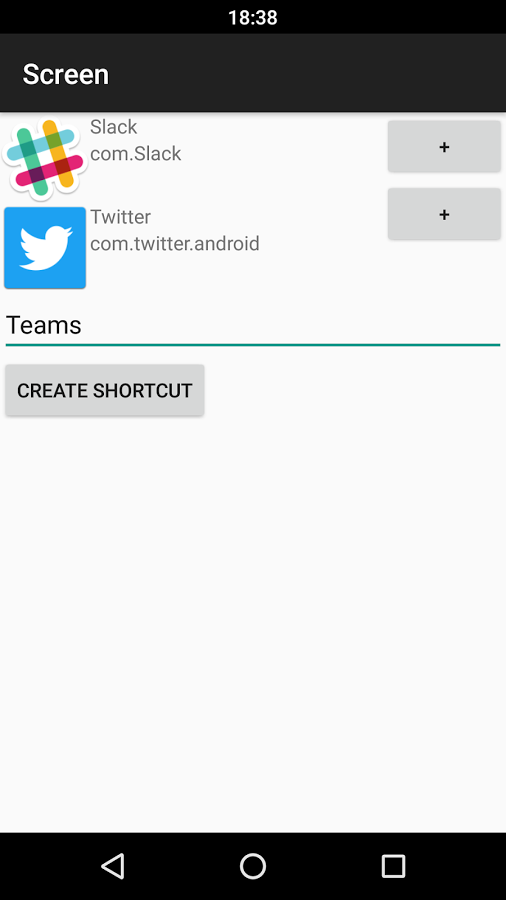The image is a portrait-mode screenshot showcasing a partially completed task within an app interface. 

At the top, a black stripe traverses the upper left and right sections, while prominently displaying the number "1838" in the center. Below this, there is a lighter black stripe with the word "Screen" on the left. Proceeding downward, the interface displays two app entries. 

The first app is "Slack," though it appears misspelled as "com.slack". Adjacent to Slack, on the left, is a distinctive hashtag logo resembling popsicle sticks arranged in green, yellow, light blue, and red colors.

The second app listed is "Twitter," formatted as "com.twitter.android". The corresponding Twitter icon appears next to it but looks unusual. Both apps' entries contain their respective package names listed beneath their icons and names. Slack is denoted as "com.slack" while Twitter is listed as "com.twitter.android".

On the right side of the screen, there's a series of buttons. A gray button with plus signs near the top, followed by an entry with "Teams" underlined in green. Below this, there's a large, eye-catching gray button with green text that reads "Create Shortcut".

The bottom section of the screenshot has a light gray background and is otherwise empty, offering a clear visual break from the rest of the content.

This detailed breakdown provides a structured and thorough description of the visual elements and layout of the screenshot.